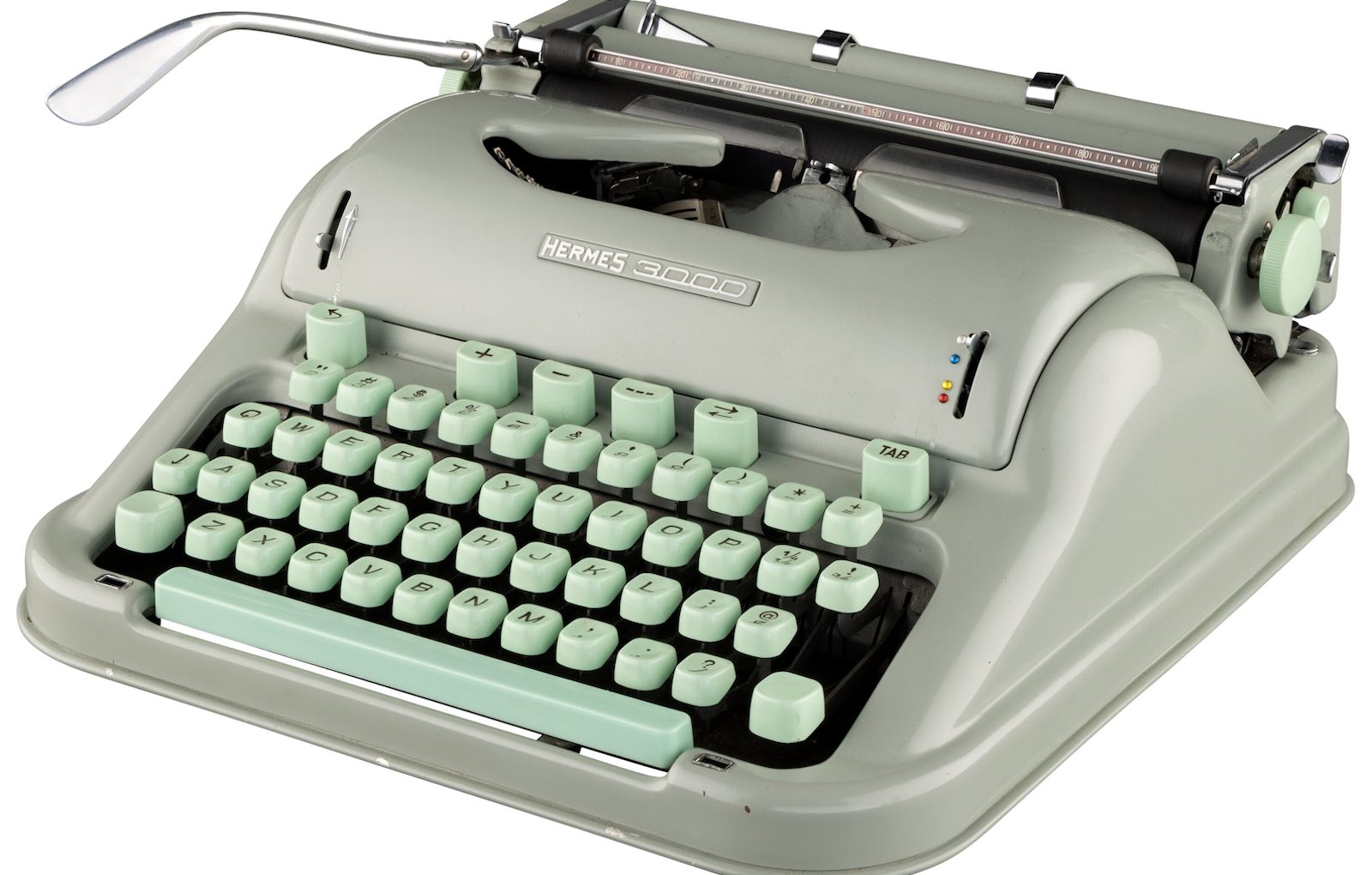This black-and-white image showcases a vintage Hermes 3000 manual typewriter, angled with the front in the lower left and the back in the upper right. The typewriter, primarily in a light bluish-gray color with metallic and reflective elements, features black, sans-serif capitalized letters on its keys, which are mounted to metal bars. Prominent on its face is the branding "Hermes" and "3000" in white text. The typewriter is equipped with a chrome handle on the left of its back, and two slits above the keyboard, with icons visible near the right slit. Its keys, designed to depress with significant pressure, and the mechanical bar for returning the page, underline its classical design. Set against a white background, the typewriter's distinctive light blue and light blue-green accents, including the roller knob, stand out, making this a striking image of a nostalgic writing tool.